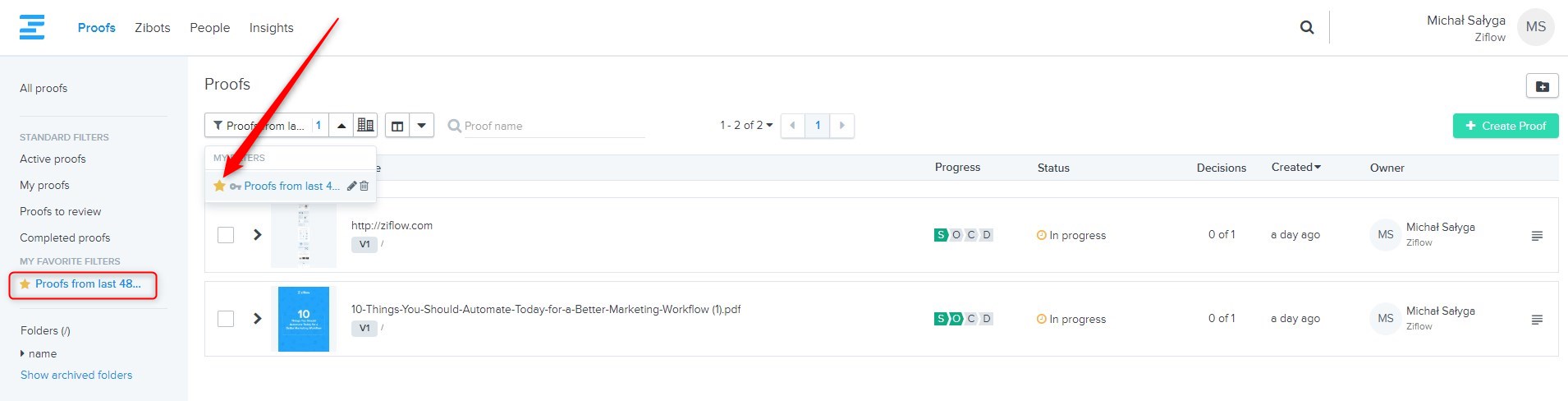**Detailed Caption:**
The image displays an interface of a professional web application, reminiscent of an email or project management account. In the top left corner, the company's logo is prominently visible. The logo features a sequence of staggered blue lines of varying lengths, alongside the text "Proofs" also in blue. Adjacent to this, the navigation menu includes options labeled "Exhibits," "People," and "Insights," all printed in a standard black font.

Centrally located, there is a search bar designed for efficient navigation. The current user, identified as Michael Salga (MS), has their account details displayed immediately below, marked with the company name "Zillow." 

On the left-hand sidebar, the user can access various categories under the "Proofs" section, which include "All Proofs," "Active Proofs," "My Proofs," "Proofs to Reveal," and "Completed Proofs." Below this is a personalized section titled "My Favorite Filters," showcasing a highlighted filter named "Proofs from the last 48 hours," denoted in blue with an accompanying yellow star.

In the main content area beneath the search bar, the filter "Proofs from the last 48 hours" is active. The screen displays project updates including: 
1. A project titled "Zillowflow.com," marked as "In Progress" with the status identifier "S," created a day ago.
2. An article "10 Things You Should Automate Today for a Better Marketing Workflow," also in progress, marked with the status "SO," and similarly created a day ago.

These details suggest a focus on recent work and active projects curated for the user.